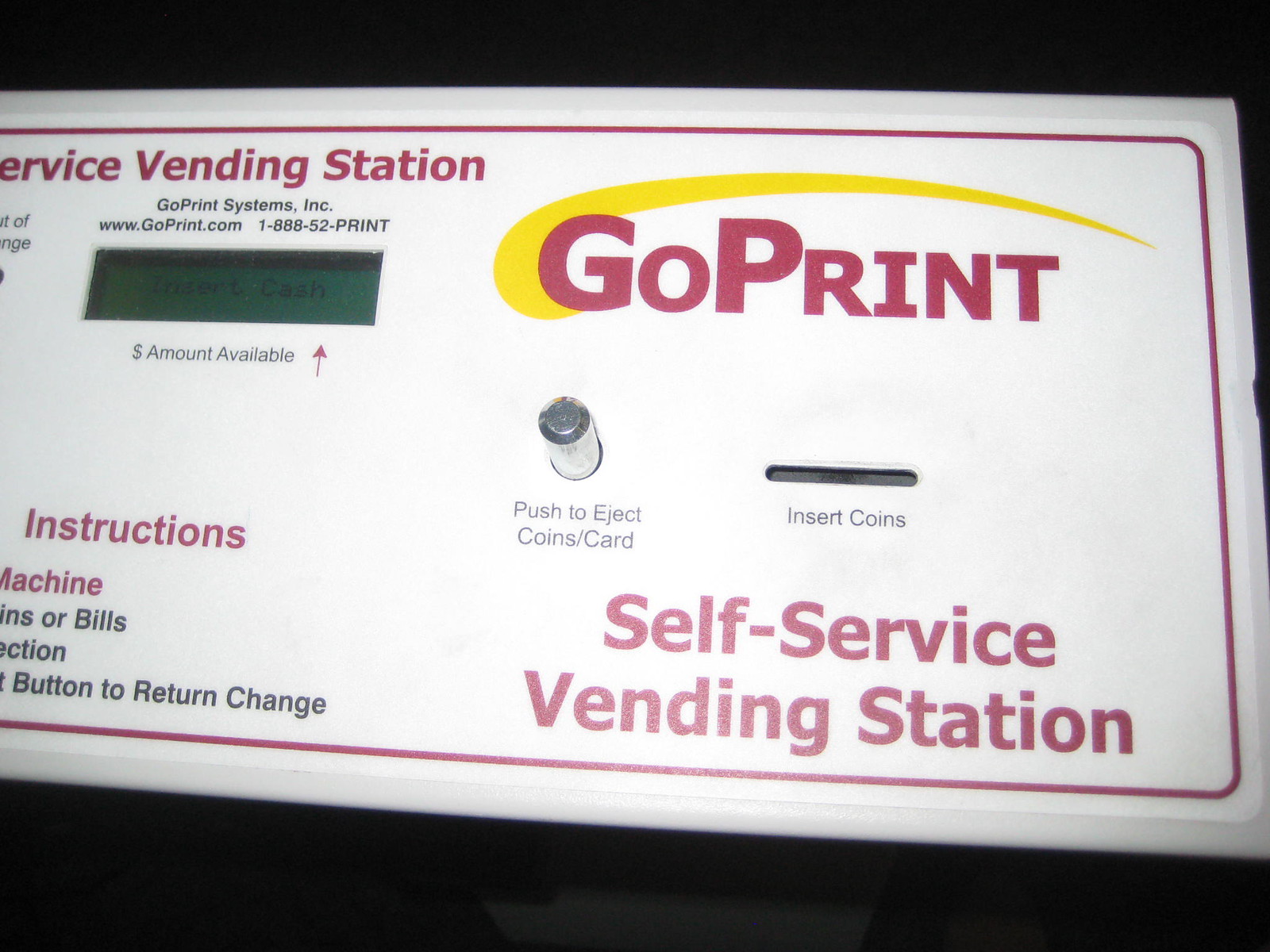This close-up photograph captures a GoPrint self-service vending machine with a sleek white design. Prominently featured at the center top is the brand name "GoPrint," styled in pink letters with a distinctive yellow swoop extending from the 'G' above the word "print." Below the GoPrint branding, the machine displays a coin slot accompanied by the instruction "insert coins" below it. Adjacent to the slot is a silver button labeled "push to eject coins/card." The right side of the machine also includes additional red text stating "self-serving vending station."

On the left, a digital screen indicates the available balance with the message "amount available in dollars," complemented by an arrow pointing to the display. Below this, further detailed instructions for using the machine are provided, though some text appears partially obscured. The machine is distinctly marked by black text at the lower left that reads "GoPrint Systems Inc., GoPrint.com, 1-800-52-PRINT," tying back to the GoPrint brand. The vending machine combines practical functionality with accessible design, making it clear and straightforward for users to operate.